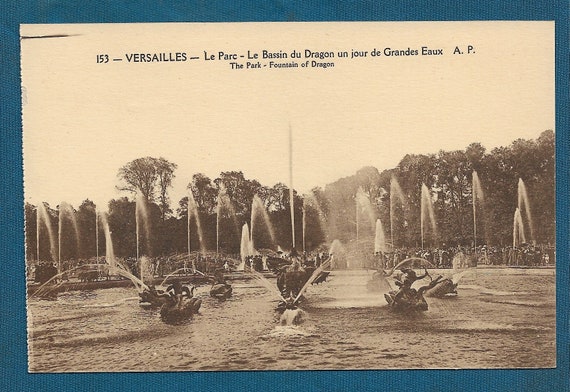The image depicts a sepia-toned, now blurred photo framed against a dark blue surface. It showcases an elaborate scene of people rowing boats on a body of water. This scene is set in front of a grand fountain adorned with dragon sculptures, with water majestically shooting upwards from the base. Surrounding the fountain are vast, towering trees under a bright, clear sky. At the top of the image, there is text in both French and English, reading, "153-Versailles, Le Parc, Le Basin du Dragon, Un Jour de Grande Aux, A.P.," which translates to "The Park, Fountain of the Dragon." The historical and picturesque elements create a vibrant yet serene tableau, though the photographic blur and sepia tone evoke a sense of nostalgia.